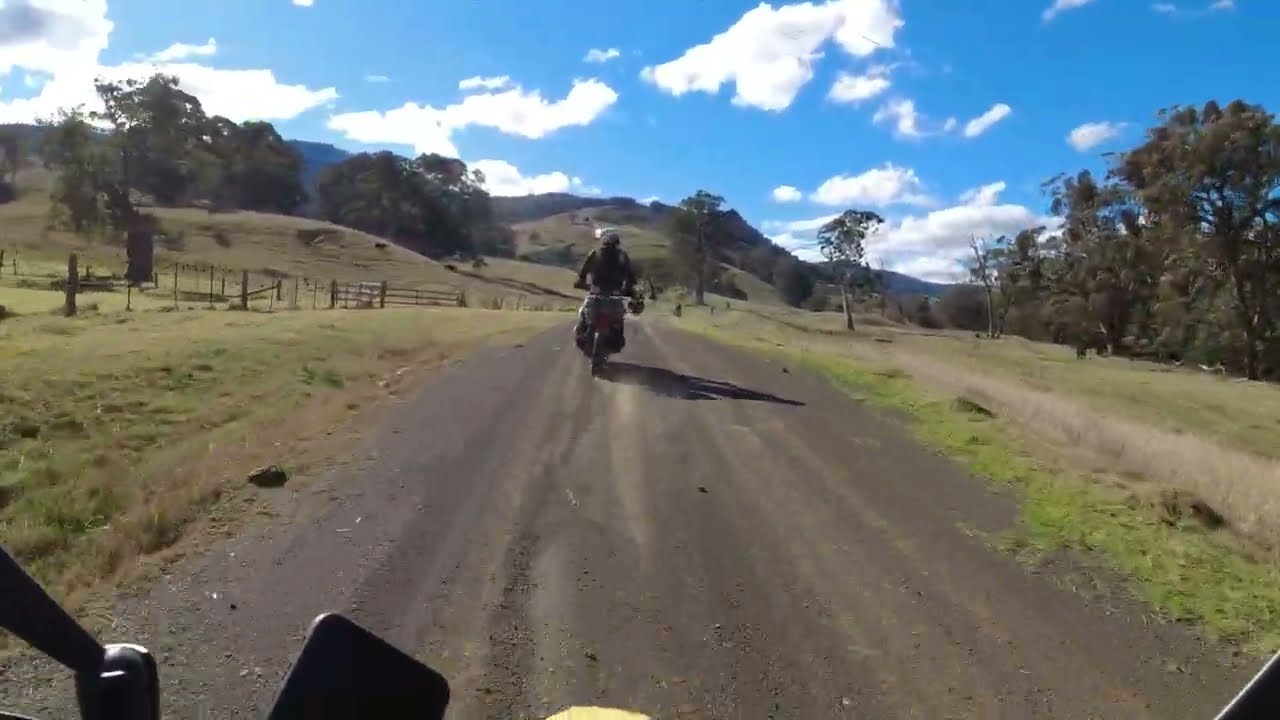This image captures a pair of motorcycle riders navigating a scenic dirt road in a rural, hilly landscape. The picture is taken from a mounted camera, likely a helmet cam or a GoPro, visible at the bottom of the frame, where you can also see part of the motorcycle’s handlebars or mirror. Approximately 20 feet ahead, another motorcycle rider, clad in a black leather jacket and an old-style helmet reminiscent of American Army gear, is leading the way. Both motorcycles appear vintage, possibly from the 40s or 50s.

The surroundings feature low-lying hills and small mountains with a mix of dry, tan areas and green fields dotted with trees, suggesting a farmland area possibly used for livestock rather than crops. A wooden fence runs along the left side, adding to the rustic atmosphere. The sky above is vibrant blue, peppered with fluffy, cotton-like white clouds, indicating a clear and sunny day. The absence of houses or other structures enhances the sense of seclusion and adventure, as the two riders enjoy their rural journey.